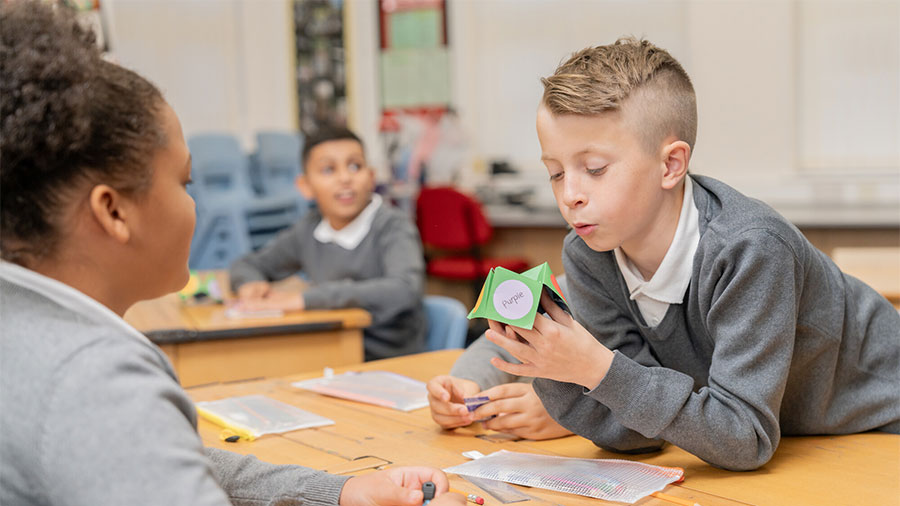In the center of this well-lit, modern classroom with off-white walls adorned with posters, stands a large, brown wooden table, pristine and free of scratches. On each side of the table sit two children in gray sweaters. On the left is a young African girl with black, curly hair tied up, intently observing a game, while on the right is a blonde-haired, white boy with an undercut hairstyle, absorbed in playing a classic paper-folded game, commonly known as a paper fortune teller. The boy is shown leaning over the table, his hands and part of his body resting on it, holding the green and yellowish paper game that features various handwritten words. Scattered on the table are numerous papers, cuttings, scales, and other crafting materials, signifying an ongoing creative activity. In the background, slightly blurred, another student is seated at a wooden desk with a blue chair, engrossed in his activity, showcasing a happy expression. Nearby, a red chair and a stack of blue chairs add to the classroom's neat and organized appeal.